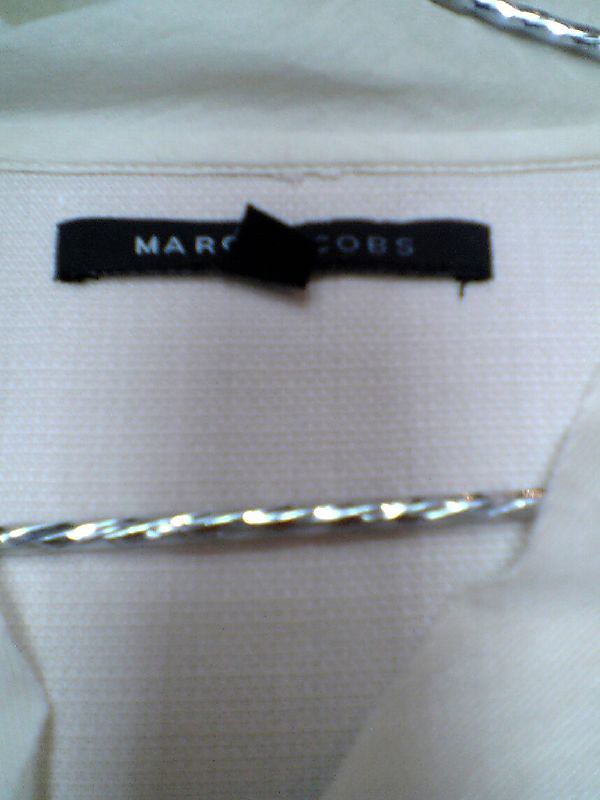This close-up, color photograph captures the inside back portion of a Marc Jacobs shirt hanging on a silver hanger. The image is slightly blurry, accentuated by the low-quality lighting that casts a cyan tint over the scene. The entire frame is filled with the textured fabric of the shirt, which is primarily white. The silver hanger, catching glints of light from above, adds a touch of reflective detail to the composition. Near the top of the image, the shirt's collar is prominently displayed. A black tag, sewn across the inside upper portion of the shirt, appears fuzzy and partially obscured, with the letters "M-A-R-C C-O-B-S" discernible despite the blur. A smaller, center tag indicating the shirt's size is flipped upwards, making part of the labeling content clear. The overall impression is a candid, impromptu snapshot that captures the essence of a Marc Jacobs garment in a raw and unpolished manner.